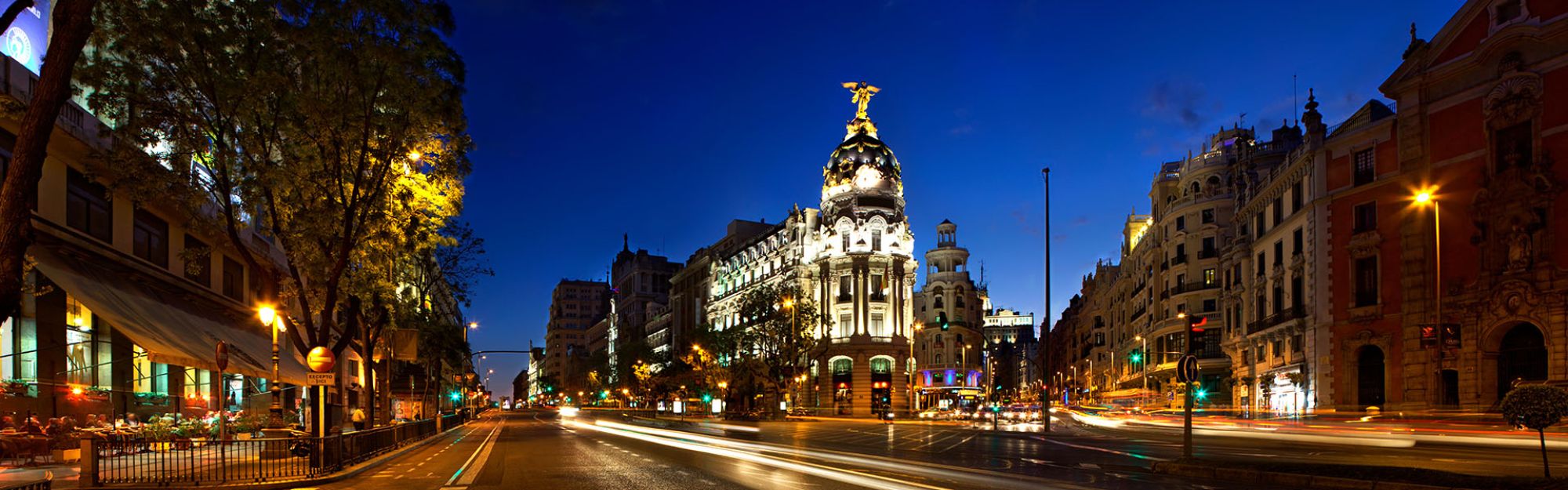This panoramic photograph, shaped like a long, thin rectangle akin to a bookmark, captures a bustling cityscape at night. Dominating the scene, a well-lit, multi-story building stands majestically in the center, glowing with white lights. The sky overhead gradates from dark to lighter blue, hinting at the twilight hour. A clear asphalt roadway runs horizontally through the middle of the image, adorned with intermittent white lane markings and a striking motion blur of headlights and taillights that hint at a time-lapse capture.

To the left, an inviting outdoor restaurant is nestled behind a short iron gate, with streetlights and illuminated trees casting a warm glow over the area. This section includes a storefront with an awning, enhancing the cozy ambiance. On the right, the streetscape transitions to more historic European-style buildings, showcasing old brick and stone facades under bright city lights. Throughout the scene, trees intermittently line the road, contributing to the picturesque urban setting. Notably, there are no visible people or stationary vehicles, adding to the serene yet dynamic night-time atmosphere.